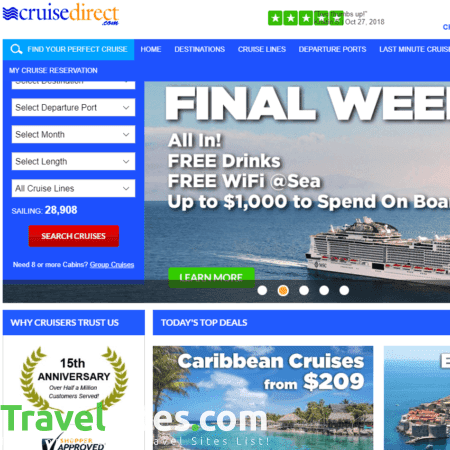The image shows the homepage of the CruiseDirect website, designed with a user-friendly interface for booking cruises. At the top of the page, "CruiseDirect" is prominently displayed, accompanied by a rating of five green stars and a "Thumbs Up" badge dated October 27, 2018. Below this is a distinctive blue band containing a light blue search bar, encouraging users to "Find Your Perfect Cruise."

The page features a bright blue background that extends to the top and sides. At the top, navigation links provide quick access to various sections, labeled "Home," "Destinations," "Cruise Lines," "Departure Ports," and a truncated "Last-Minute Cruise." On the left side, "My Cruise Reservation" is displayed, along with several drop-down menus for selecting departure port, month, length, and cruise lines. Users can refine their search with these options, leading to a red "Search Cruises" button with white font for initiating a query. 

The main section also includes a note about booking eight or more cabins for group cruises, underlined for emphasis. Centrally located is a promotional banner with a partially visible message that emphasizes the final week of a special offer, which includes free drinks, free Wi-Fi at sea, and up to $1,000 to spend onboard.